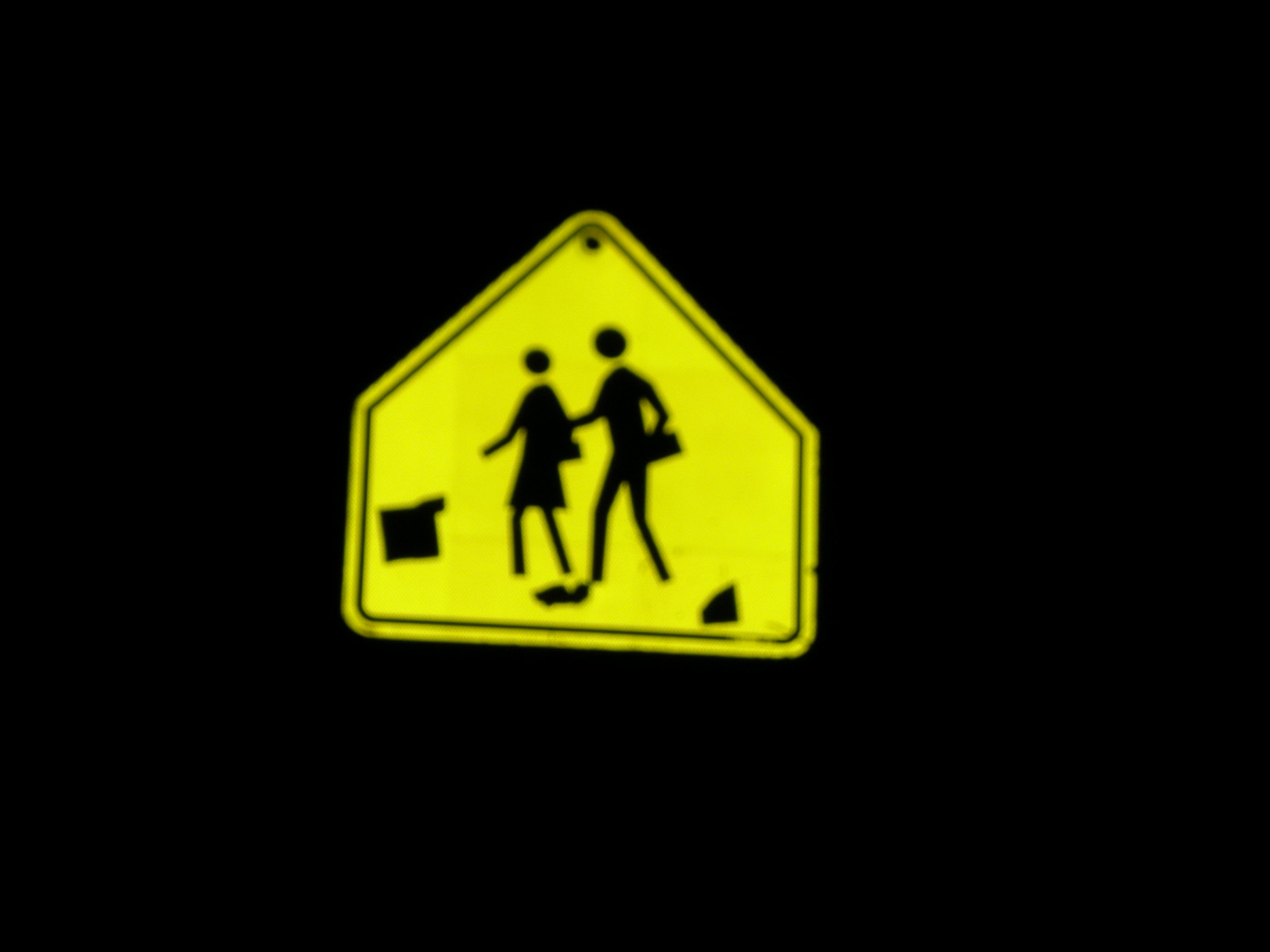This photograph, though blurry, features a distinctive yellow pentagonal street sign set against an entirely black background. Slightly off-center to the left, the sign has a thin black border and a small hole at its peak. The main focus of the sign is a simplified diagram of two black stick-figure people. The person on the right is taller and appears to be holding an object, resembling a briefcase, with one arm while touching the shorter individual on their left, who is characterized by a dress, potentially indicating a woman. Below the figures are a series of geometric shapes: a black square near the bottom, accompanied by a blob-like shape and a sideways triangle to the right.